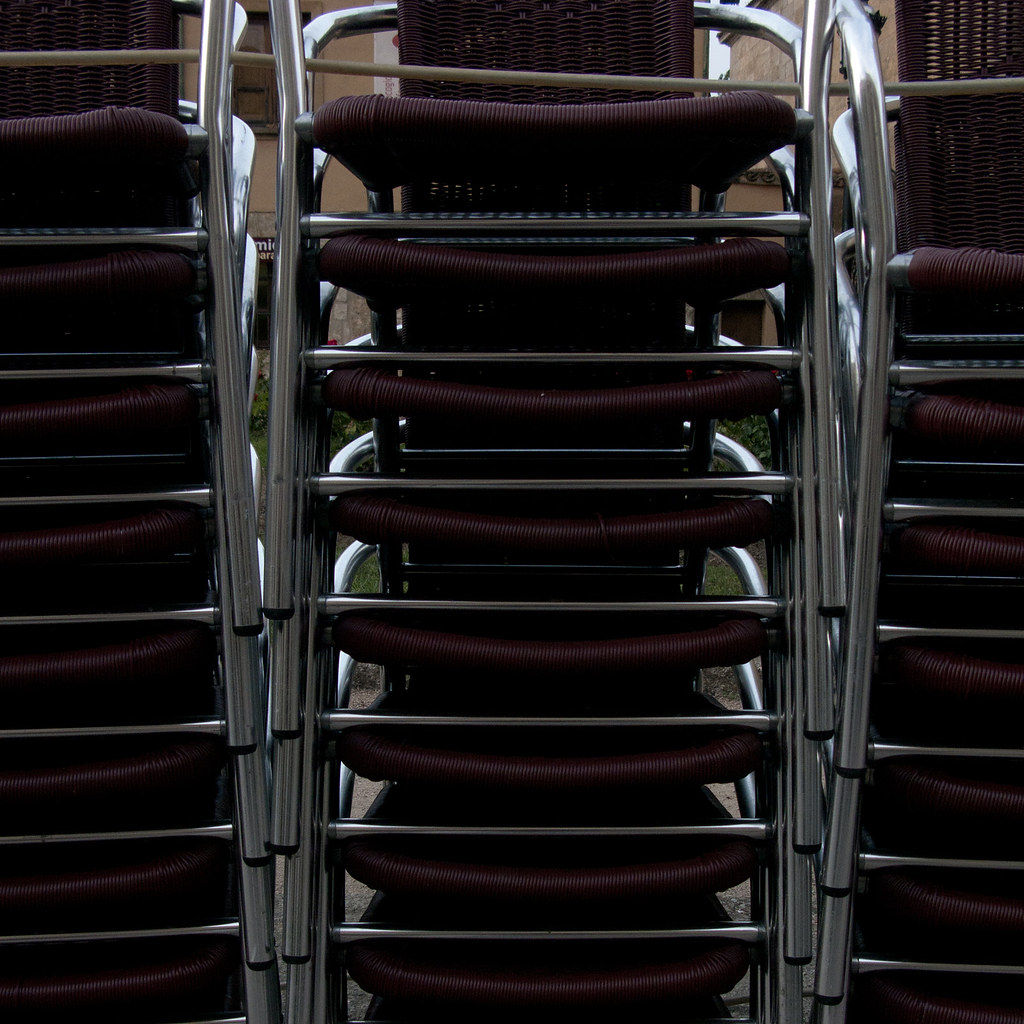This photograph depicts three tall stacks of chairs made from a dark maroon wicker-like material, tightly woven, giving a consistent appearance. Each stack comprises approximately 8 to 10 chairs, with the central stack fully visible and occupying the majority of the frame, and the flanking stacks partially visible. The chairs feature sturdy, silver metal frames with tubular arms and legs, and the legs have black rubber stoppers. The tops of each stack are secured with a wooden pole or cable, likely to prevent them from toppling over. The scene appears to be outdoors, possibly in a backyard or on a patio, as suggested by the visible grass, shrubbery, and a light brown building with dark brown windows in the background. Some red flowers and a concrete walkway can also be glimpsed through the gaps between the chairs. The overall composition emphasizes the orderly yet secure arrangement of the chairs against the natural backdrop.